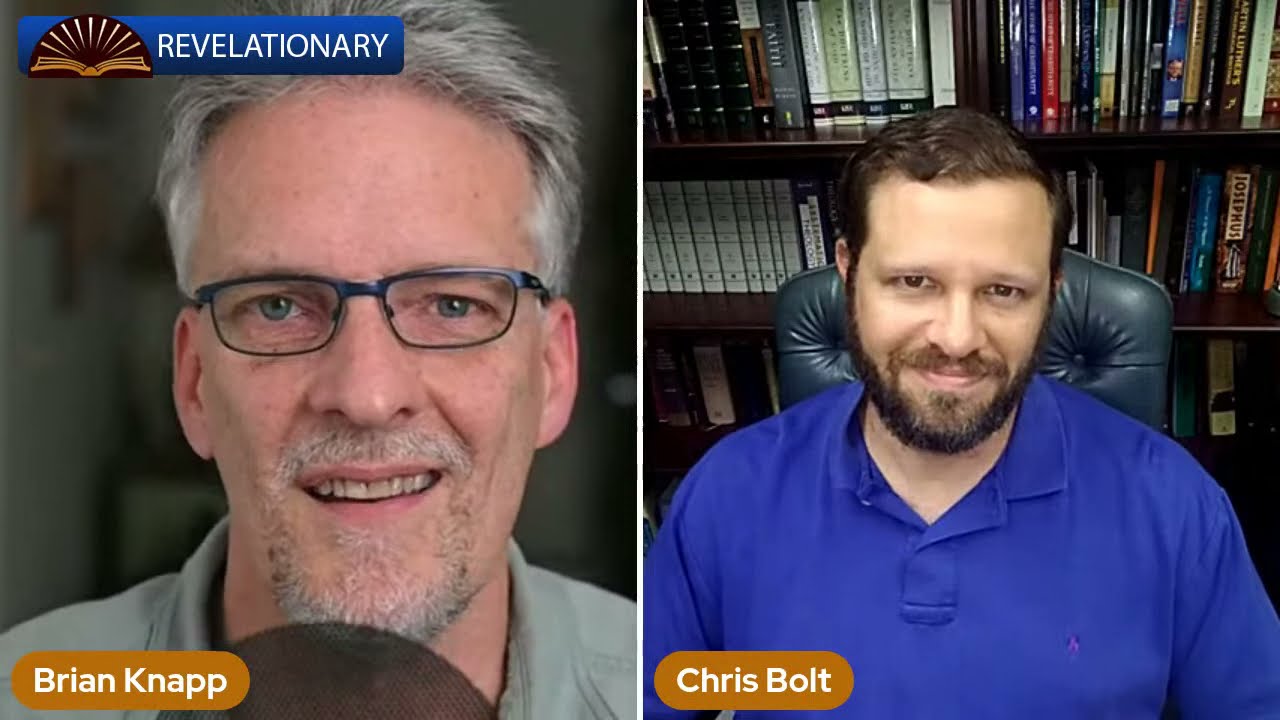The image appears to be a still from a podcast or TV show featuring two men in a split-screen format from two separate locations. On the left, the screen displays a photograph of Brian Knapp, a white man with grayish-silver hair, blue-green eyes, and black-framed glasses, slightly smiling. In the upper left corner of this section, a blue rectangle with the word "Revelationary" in white letters and a golden open book icon emitting rays is prominently featured. The background is blurry and grayish, keeping the focus on Brian. Underneath his image, his name, "Brian Knapp," is displayed. On the right side, another man, Chris Bolt, is sitting in a blue chair with a bookshelf filled with books behind him. Chris, who has brown hair, a mustache, and a beard, is also almost smiling and is wearing a blue polo shirt. His name, "Chris Bolt," is shown at the bottom left corner of his part of the image. The setup suggests a conversation between the two men, possibly via a video call.